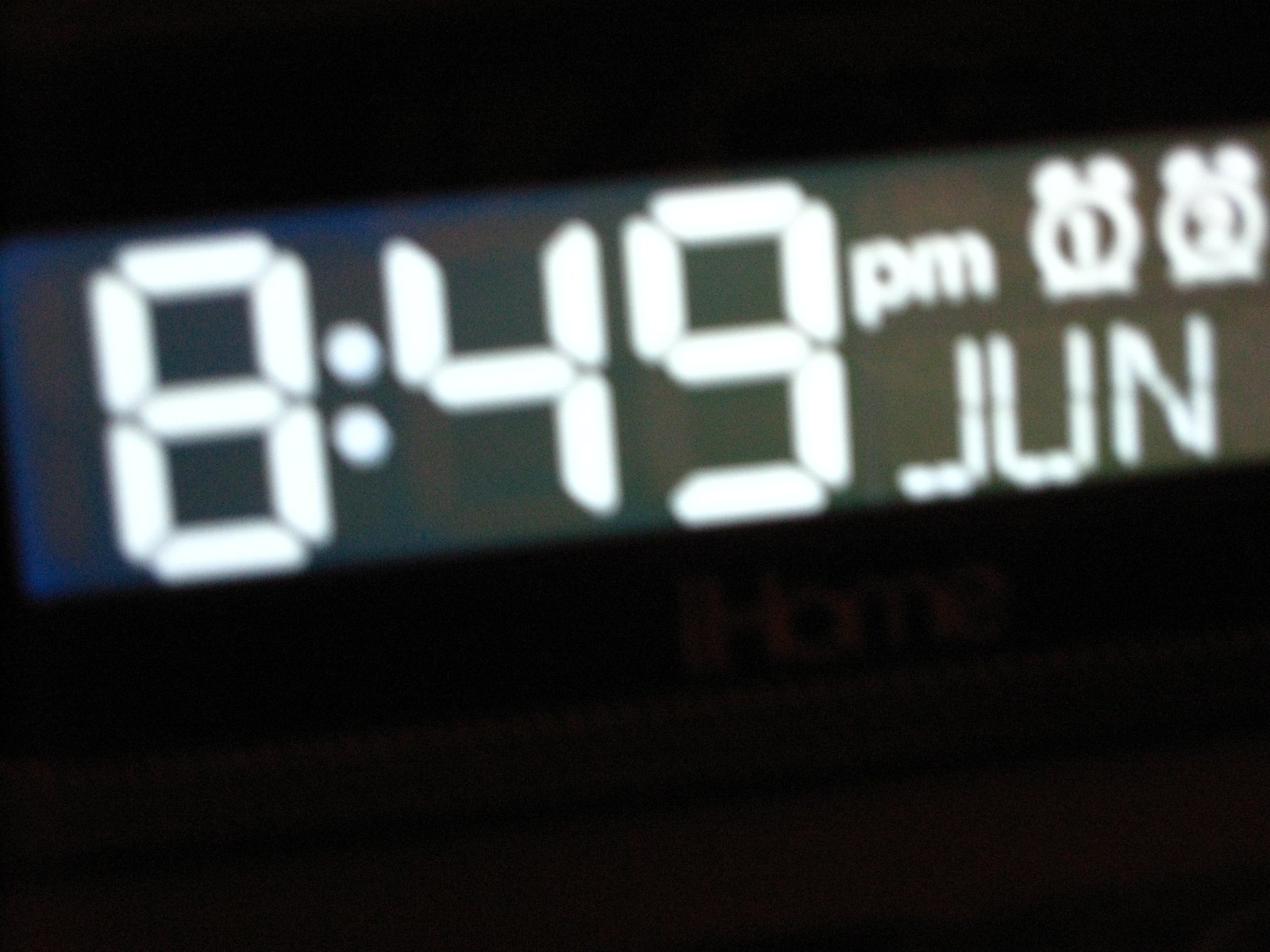A dimly lit digital clock display shows the time as 8:49 PM and the date as June. The display features the typical geometric, round-shaped font, characterized by rectangles pieced together to form the letters and numbers. In the upper right corner, there are icons of two small clocks labeled '1' and '2,' indicating the presence of two set alarms. Although the image is slightly blurry, the essential details remain discernible. The overall scene appears to be captured in a dark room or at nighttime, making the bright display of the digital clock stand out.